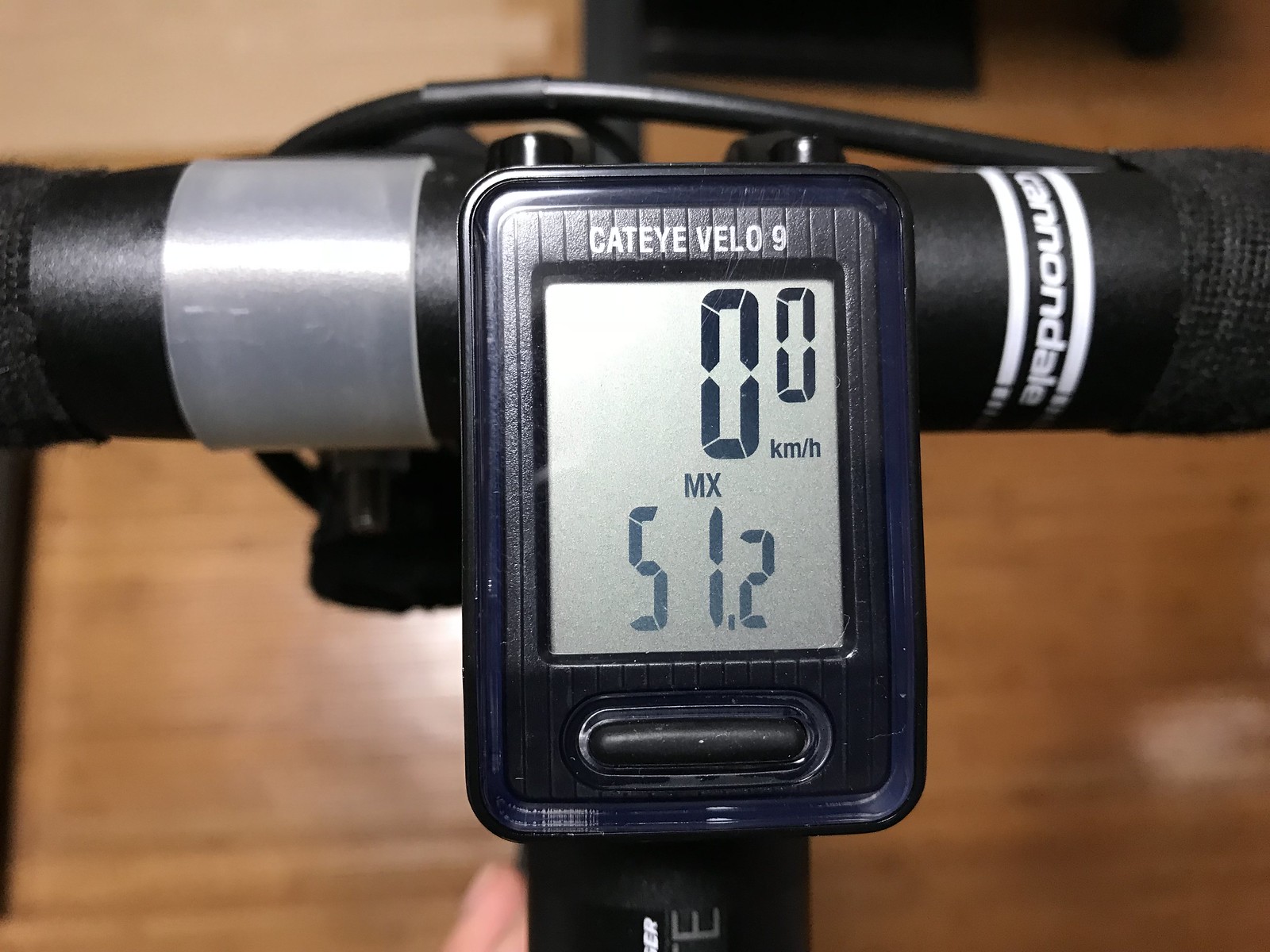This indoor photograph showcases a bicycle or exercise bike, predominantly illuminated by overhead lighting which casts a focused glow on the subject. The background reveals a slightly out-of-focus wooden floor, boasting a honey-colored, light brown hue, paired with a cream-painted wall. A black object emerges from the top right corner of the image, adding to the composition. The bike's black handlebars, positioned either to one side or centrally, are equipped with visible brake cables. A silver piece of tape, accompanied by a white "Cannondale" brand name, adorns one of the bars. The centerpiece of the photograph is a CatEye Velo 9 digital display, prominently showing "kilometers per hour" with an MX reading of 51.2, mounted on a horizontal bar descending from the bike’s frame.